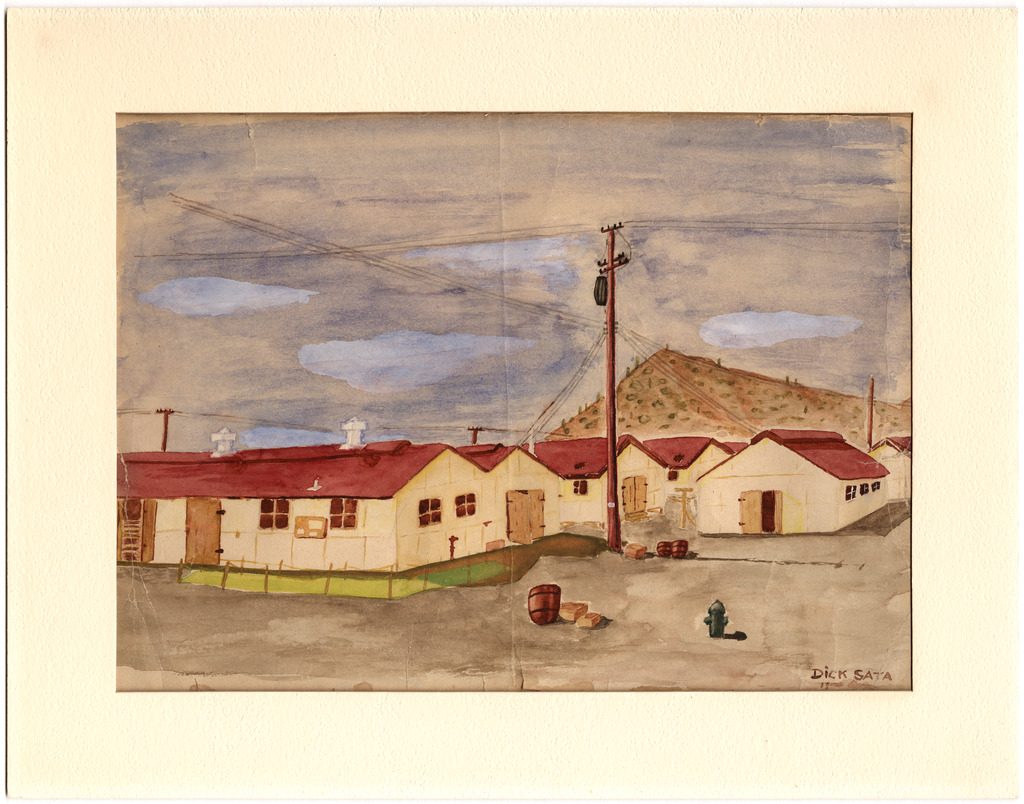This is a framed watercolor painting, mounted with an ivory-colored mat. The artwork depicts a desert environment featuring white, single-story buildings with red roofs and brown doors. The buildings, arranged in two rows, have a uniform appearance, almost reminiscent of military barracks, with windows and distinctive red roofs. On the foremost building to the left, there are cylindrical or conical metal ventilators on the roof. Right of center stands a wooden telephone pole with black wires extending in both directions, connecting to the buildings. A green fire hydrant is located in the lower right corner. The foreground of the painting is characterized by grayish dirt. In the background, a large sandy hill dotted with green bushes is set against a cloudy, gray sky with occasional blue patches. A dark brown barrel is also visible. The painting is signed "Dixada" or "Dick Sata" in the lower right corner.